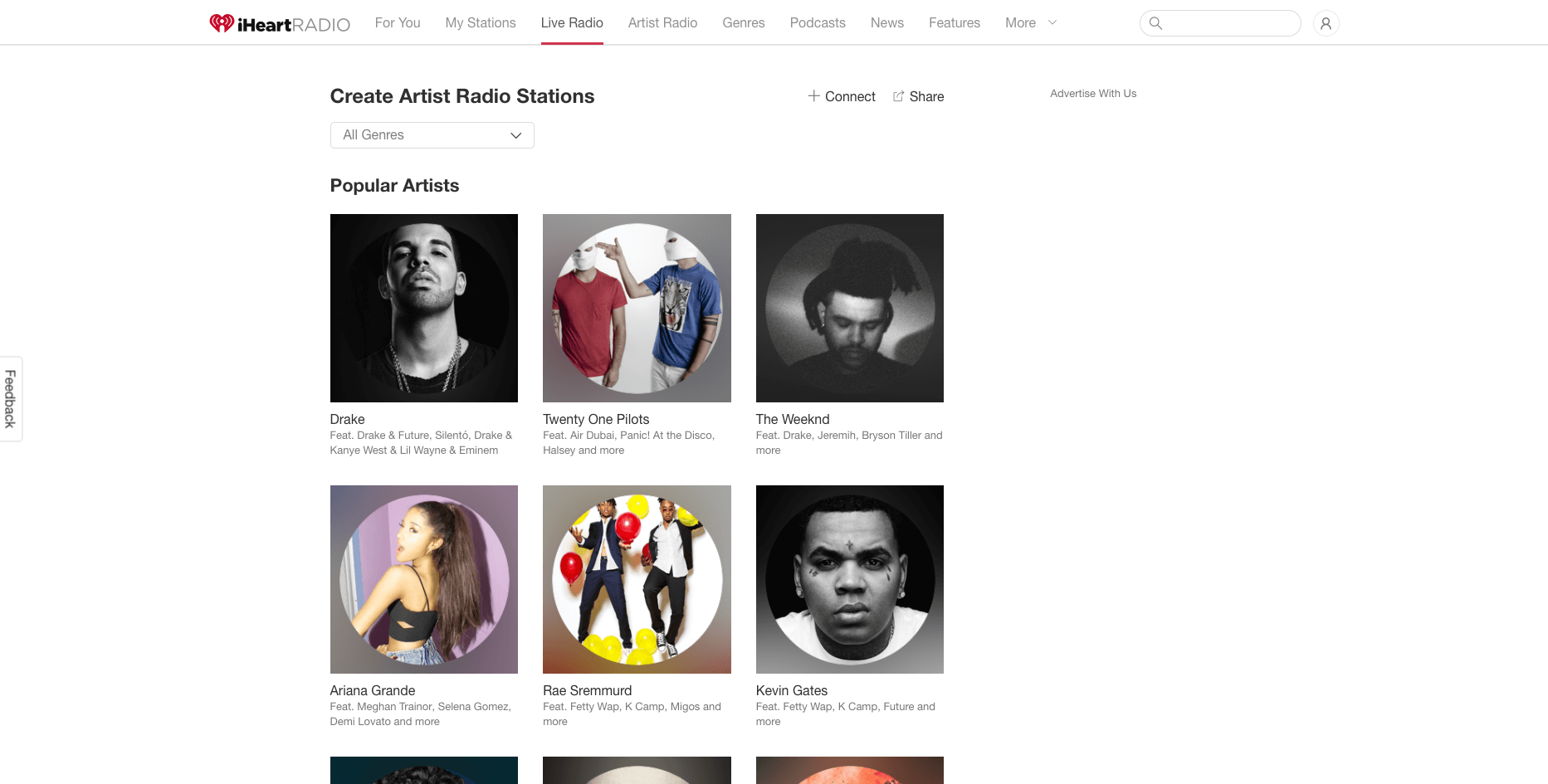The image showcases an I Heart Radio interface against a white background. At the top, a broken red heart icon is accompanied by the "I Heart Radio" text. Below it, tabs label "For You," "My Services," and "Live Radio," with "Live Radio" underlined in red. Additional tabs include "Arts Radio," "Genres," "Podcast," "News Feature," and "More," with a small gray down arrow indicating a dropdown menu. A prominent search box is present alongside a circular icon featuring a stylized person. 

A grey separator line below highlights the text, "Create Artist Radio Stations," and there's a button labeled "All Genres." Adjacent buttons include a "+" symbol representing "Connect" and a "Share" option. Partially obscured text suggests instructions or options, though some words are illegible. 

Below these, six images represent "Popular Artists," including names like Ariana Grande, Rae Sremmurd, and Kevin Gates, each accompanied by their respective pictures. The top portions of three additional images and artist names are barely visible at the bottom of the interface.